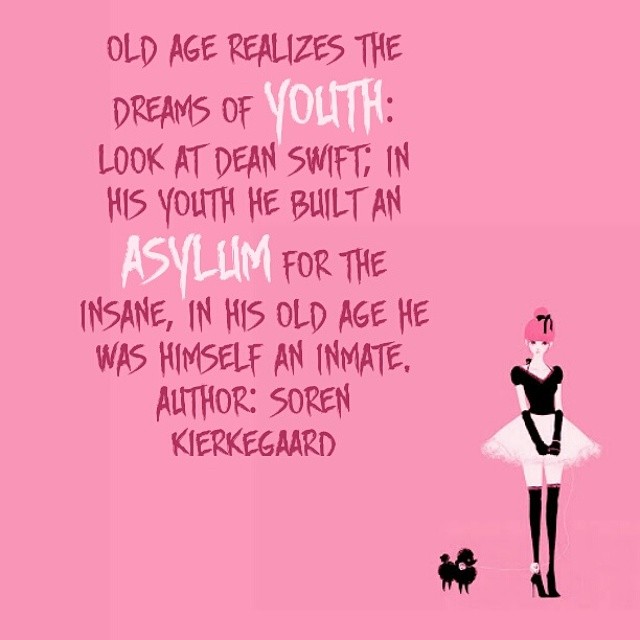This image resembles a greeting card or an internet meme and features a violently pink background. The layout is vertical in size and shape. On the bottom right, there's an illustration of a girl dressed somewhat like a ballerina, though with unique attire: she is white, wearing a black top, black gloves, a white skirt, long black leggings, and black high heels. To her left stands a black poodle. The image contains text that runs from top to bottom in stylized red and white fonts. Two words, "youth" and "asylum," are particularly prominent in white. The text reads, "Old age realizes the dreams of youth. Look at Dean Swift. In his youth, he built an asylum for the insane. In his old age, he himself was an inmate. Author Soren Kierkegaard."